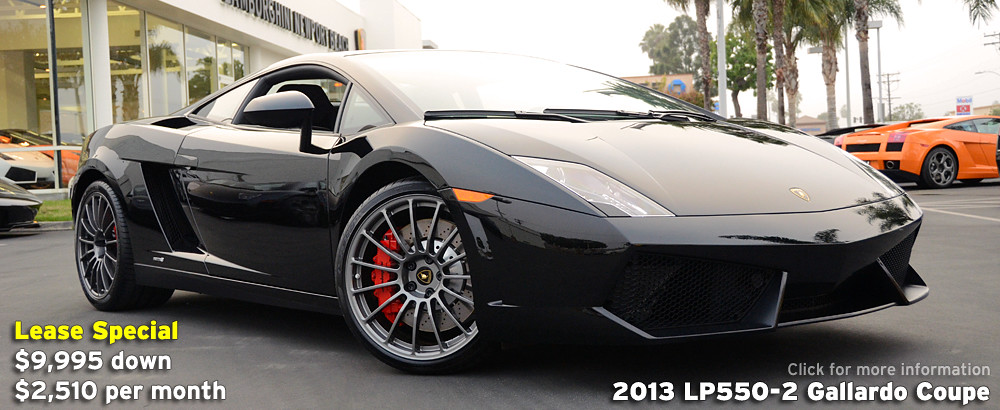A stunning, high-resolution photograph captures an advertising scene outside a luxury car dealership. The primary focus is a sleek, black 2013 Lamborghini LP550-2 Gallardo Coupe, detailed with disc brakes featuring red calipers, parked prominently in front of the dealership. Directly to the right of the black car, an eye-catching orange sports car adds a pop of vibrant color to the foreground, while another orange vehicle can be seen inside the elegantly lit showroom. The background features tall palm trees, indicating a location possibly in Florida or California, under a gray, overcast sky interspersed with telephone poles. Over the dealership building, a sign reads "New or Used," hinting at the dealership's offerings. Bold yellow text on the lower left announces a "Lease Special," with details in white stating "$9,995 down, $2,510 per month." The bottom right corner directs viewers to "Click for more information," on the 2013 LP550-2 Gallardo Coupe, underscoring the luxurious and affluent vibe of the entire scene.